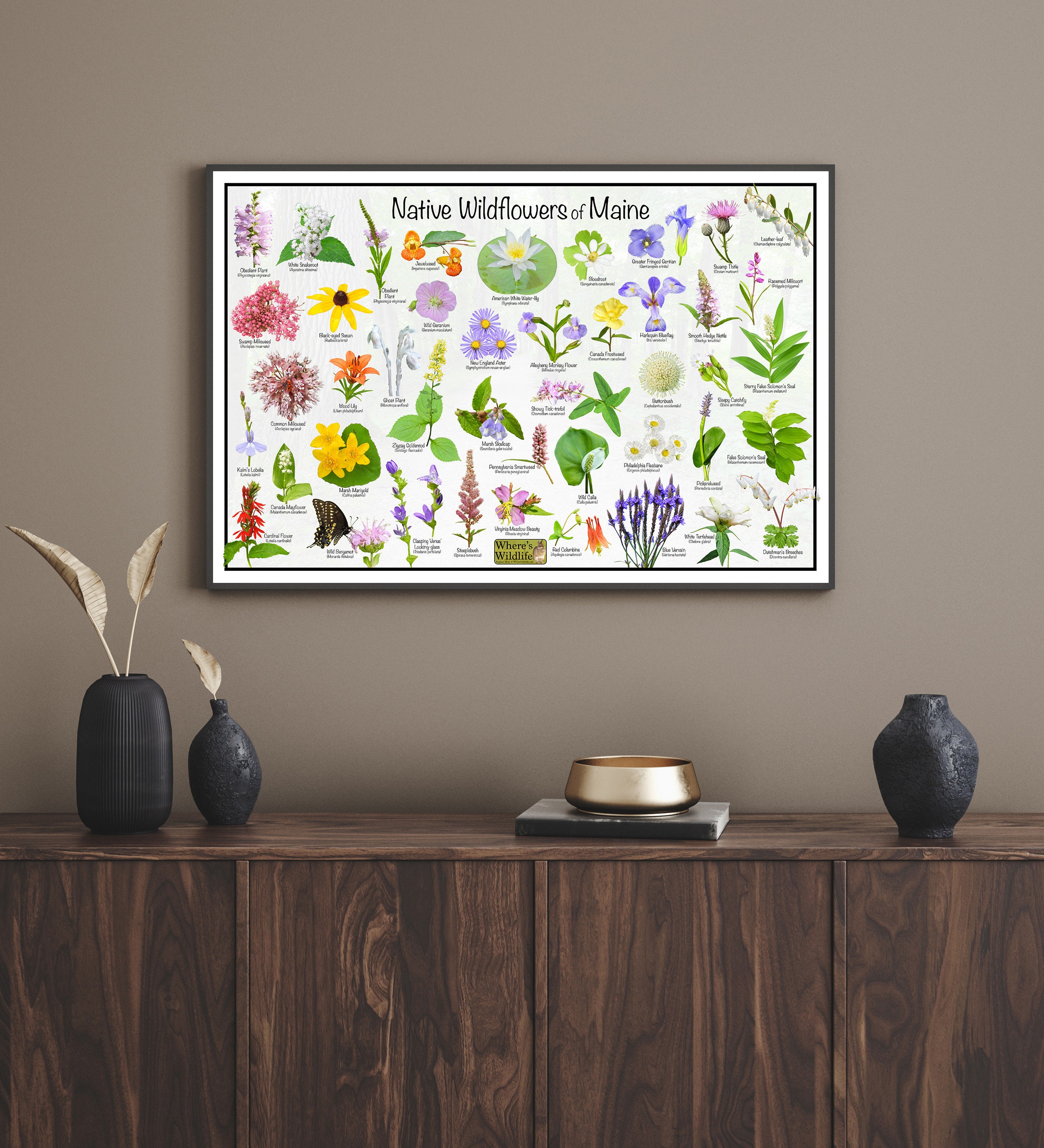The image captures a cozy living area featuring a medium-gray, tannish-gray wall adorned with a large, framed poster titled "Native Wildflowers of Maine." The poster, in a black frame with a white background, showcases approximately 40 different types of colorful flowers, including yellow, orange, red, pink, purple, and violet blooms, alongside various green foliage. Beneath each flower illustration is illegible text, presumably naming the species. Below the poster stands a sleek, dark wooden sidebar or cabinet without drawers, featuring doors on the front. On top of the furniture are three elegant black ceramic vases; two contain pale tan, dried leaves, while the third remains empty. Additionally, the vignette includes a metallic gold bowl placed atop either a book or a square slab of marble, adding a stylish accent to the display.